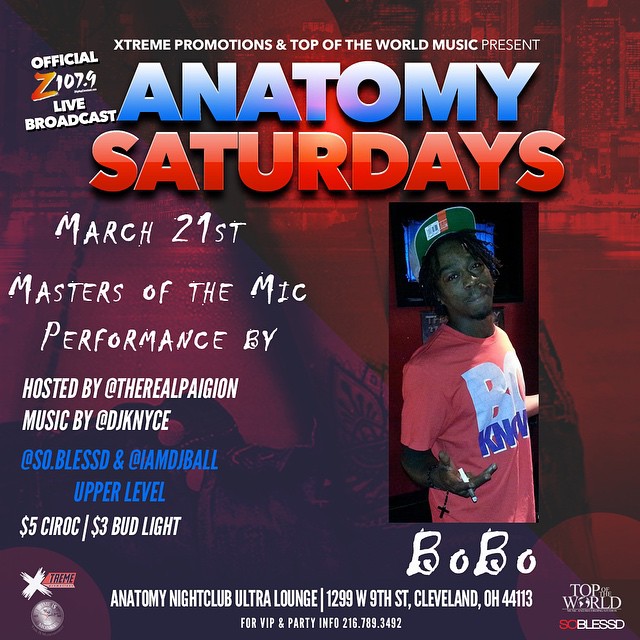The image is a detailed advertisement or flyer for a music event titled "Anatomy Saturdays." At the top, the header reads "Extreme Promotions and Top of the World Music Present" in white text, with "Anatomy" in bold blue uppercase letters and "Saturdays" in matching bold red uppercase letters. The upper left-hand corner features "Official Z 107.9 Live Broadcast." 

Beneath the title, to the right, is a photo of an African-American man wearing a black cap, red t-shirt, and possibly holding a cigarette. He has dreadlocks and is identified as "Bobo" in white graphic font beneath his image. To the left of the photograph, the poster details the event specifics: "March 21st," "Masters of the Mic," "Performance by," "Hosted by @TheRealPagan," and "Music by @DJKNice."

Additional information includes drink specials—five dollars for Ciroc and three dollars for Bud Light—in white text. The bottom of the flyer provides the event venue information: "Anatomy Nightclub Ultra Lounge, 1299 W 9th Street, Cleveland, OH 44113," and a contact number "For VIP and party info: 216.789.3492." Several sponsor logos are also displayed at the bottom. The background of the flyer is burgundy adding a rich backdrop to the vibrant details.